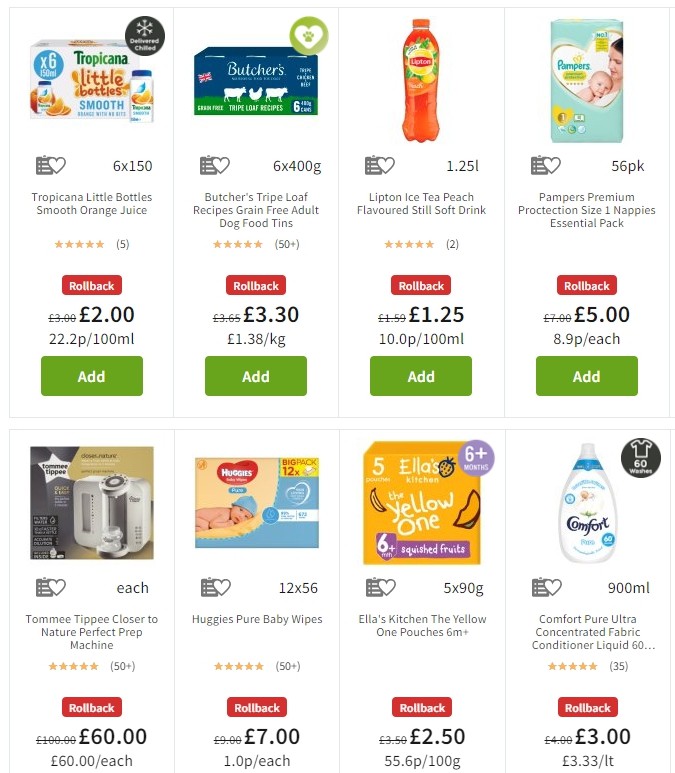Screenshot of an e-commerce webpage displaying a selection of eight diverse products, each marked with a price rollback offer and an option to add to the cart. The first item is Tropicana Smooth Orange Juice in little bottles, discounted from €3 to €2. Next, there's Butcher's Tripe Loaf Recipes grain-free adult dog food tins, reduced from €3.65 to €3.30. Following that, Lipton Iced Tea Peach Flavored Still Soft Drink is marked down from €1.59 to €1.25. Each of these three items boasts a 5-star rating.

Further down, Pampers Premium Protection Size 1 Nappies Essential Pack is on sale from €7 to €5. Also listed is the Tommee Tippee Closer to Nature Perfect Prep Machine, receiving 5-star reviews, with a significant price cut from €100 to €60. Huggies Pure Baby Wipes, also rated 5 stars, are reduced from €9 to €7. 

Additionally, Ella's Kitchen 'The Yellow One' pouch for 6 months and older infants is now €2.50, down from €3.50. Lastly, Comfort Pure Ultra Concentrate Fabric Conditioner Liquid is available for €3, reduced from €4. Each item includes a prominent 'Add to Cart' button for easy shopping, highlighting the ease and convenience of purchasing discounted, highly-rated products.